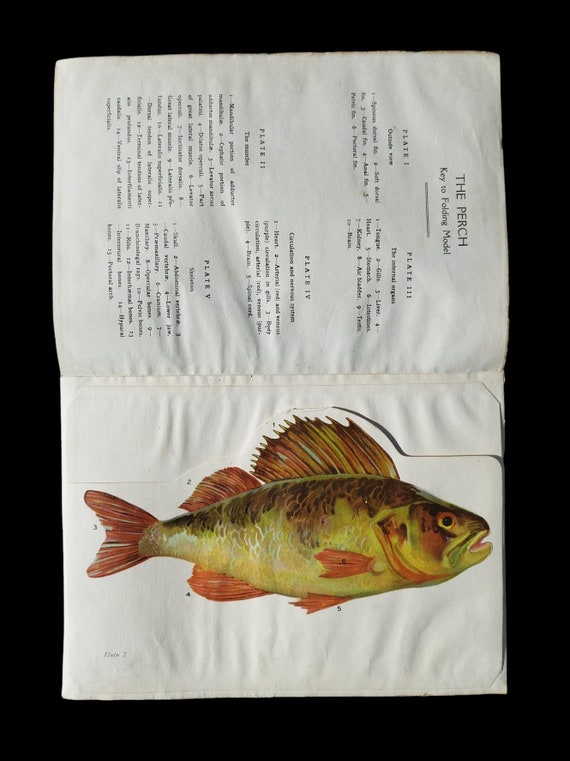The image portrays an open book with slightly rippled, white pages, possibly indicating water damage. The left-hand page features a detailed illustration of a fish, identified as a perch, with a notable high sail dorsal fin and a second shorter dorsal fin. Its coloration includes brown scales on top, yellow scales on the bottom, and multiple orange fins, including an orange tail fin. The fish has a black dot for an eye and an open mouth revealing a pink interior. Two yellow fins are located underneath its body towards the front. The fish illustration is printed on a flap that precisely follows its contours, suggesting it can be folded over. Beneath the fish illustration, the white page's background contrasts against a completely black backdrop. The right-hand page, printed in black text, is oriented vertically and reads "The Perch Key to Folding Model" at the top, followed by a gray line and several paragraphs of text organized in columns.